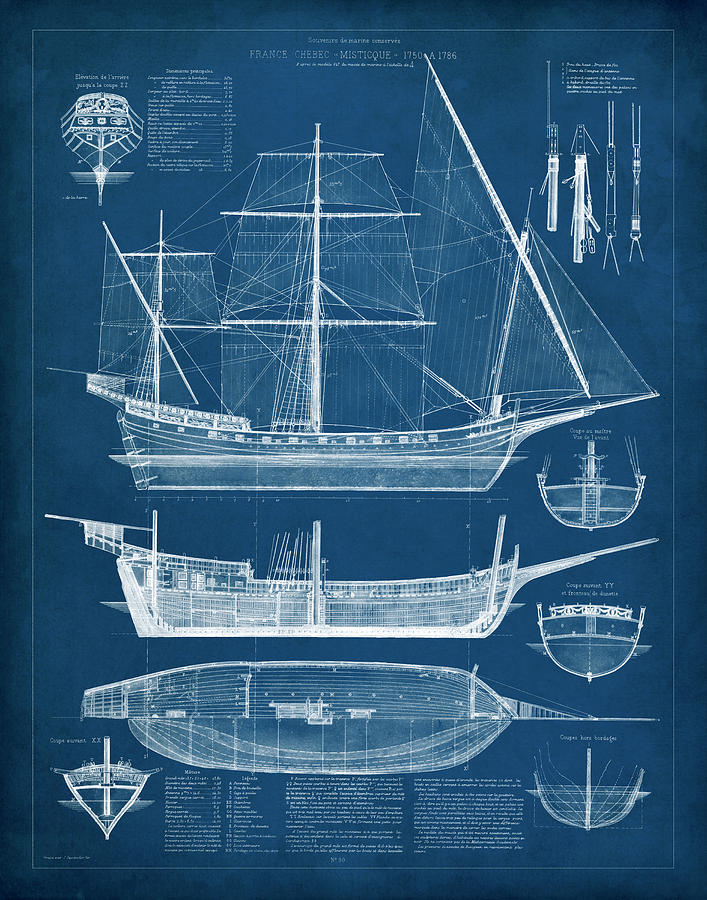The image is a detailed blueprint of a ship on dark navy-blue paper, with all drawings and writings in white. At the very top, the text reads "France CHESEC Mystique 1750 - 1786." The blueprint is laid out in a poster format with a portrait orientation. The ship is depicted from various angles: in the upper middle, there's a large side view showing its three masts, each with multiple sails, including a set of triangular sails on the right. Below this central image, the ship is illustrated without sails, emphasizing the structure of the vessel. At the bottom, there are sections showing the top and bottom halves of the ship. Additionally, on the right side of the poster, there are three more detailed views, presenting the front and back angles of the ship. This meticulous layout captures the comprehensive design and complexities of the maritime vessel from the era.